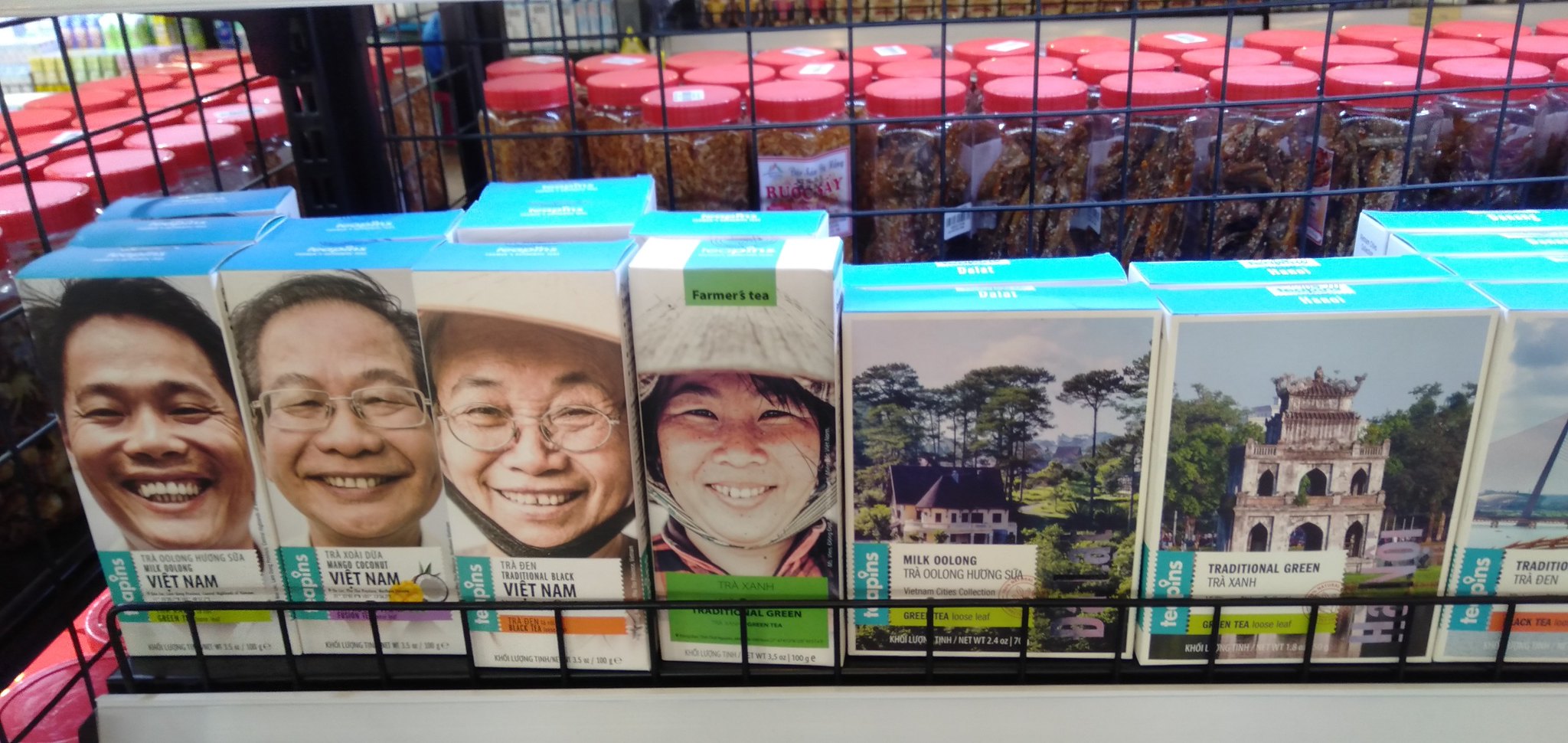The color photograph showcases a store display featuring a variety of Vietnamese tea presented on a black wire rack. At the forefront, several vibrantly designed tea boxes are neatly arranged. 

- The first box, labeled "Milk Oolong Vietnam," features a cheerful young Asian man beaming broadly.
- Next, the "Mango Coconut Vietnam" box depicts an older Asian man with glasses, also smiling warmly.
- Following that is "Traditional Black Vietnam," showcasing an elderly woman with glasses and a hat, grinning gently.
- The "Traditional Green Farmer's Tea" box displays a joyful young woman, similarly adorned with a hat.

Further down the rack, two larger boxes boast scenic landscape images:
- One box, marked "Milk Oolong Green Tea Loose Leaf Vietnam City's Collection," displays a tall house with a black roof, surrounded by towering trees.
- The other, labeled "Traditional Green Green Tea Loose Leaf," features a serene white stone temple.

Additionally, a partially visible box to the right suggests more offerings. In the background, numerous plastic containers with red lids, filled with unknown substances, are stacked on shelves. The image is wider than it is tall, capturing an exhaustive view of the vibrant tea selection and bustling store ambiance.